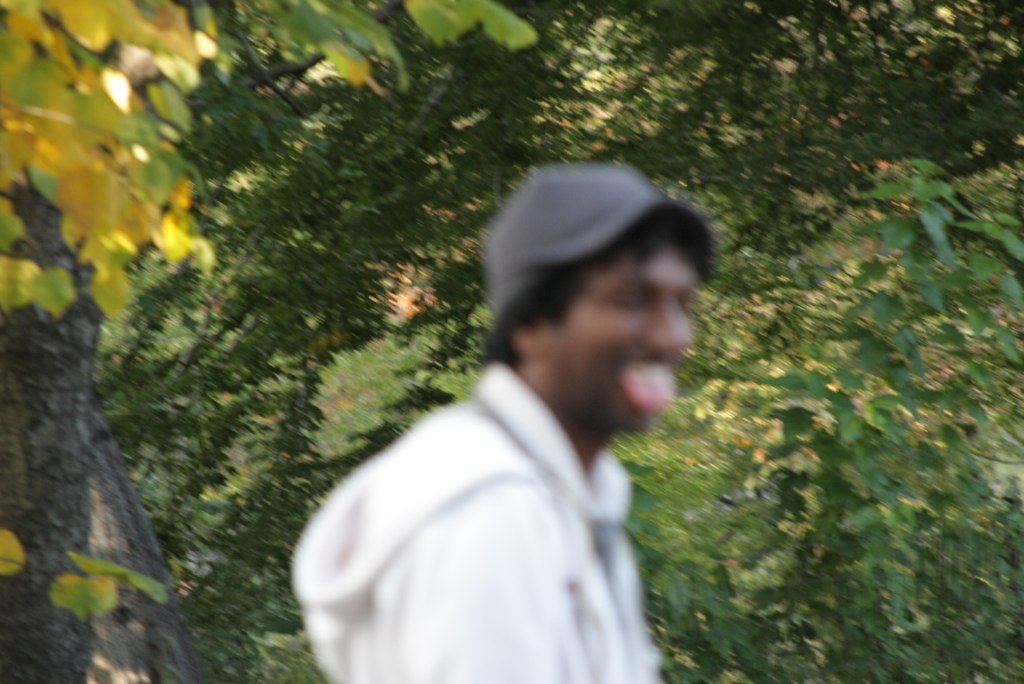In this photograph, the central focus is on a young black man smiling at the camera with his tongue slightly sticking out. He is positioned so that we see him from his right side, capturing only the upper part of his body from his bicep up. He wears a light gray hat atop short black hair and a bright white hooded sweatshirt. His eyes appear to be closed, emphasizing his playful expression. 

The background is densely filled with a variety of plant life. Behind him, tall tree branches, vines, and various plants create a wall of greenery, predominantly dark green in hue. To the left of the image, we observe leaves that range from bright yellow to green, illuminated by light filtering through. A charcoaled tree bark also runs down the left side, adding a darker element to the vegetation. Despite the general blurriness of the photo, the background details provide a rich, natural setting that emphasizes the man's joyful presence in the frame.